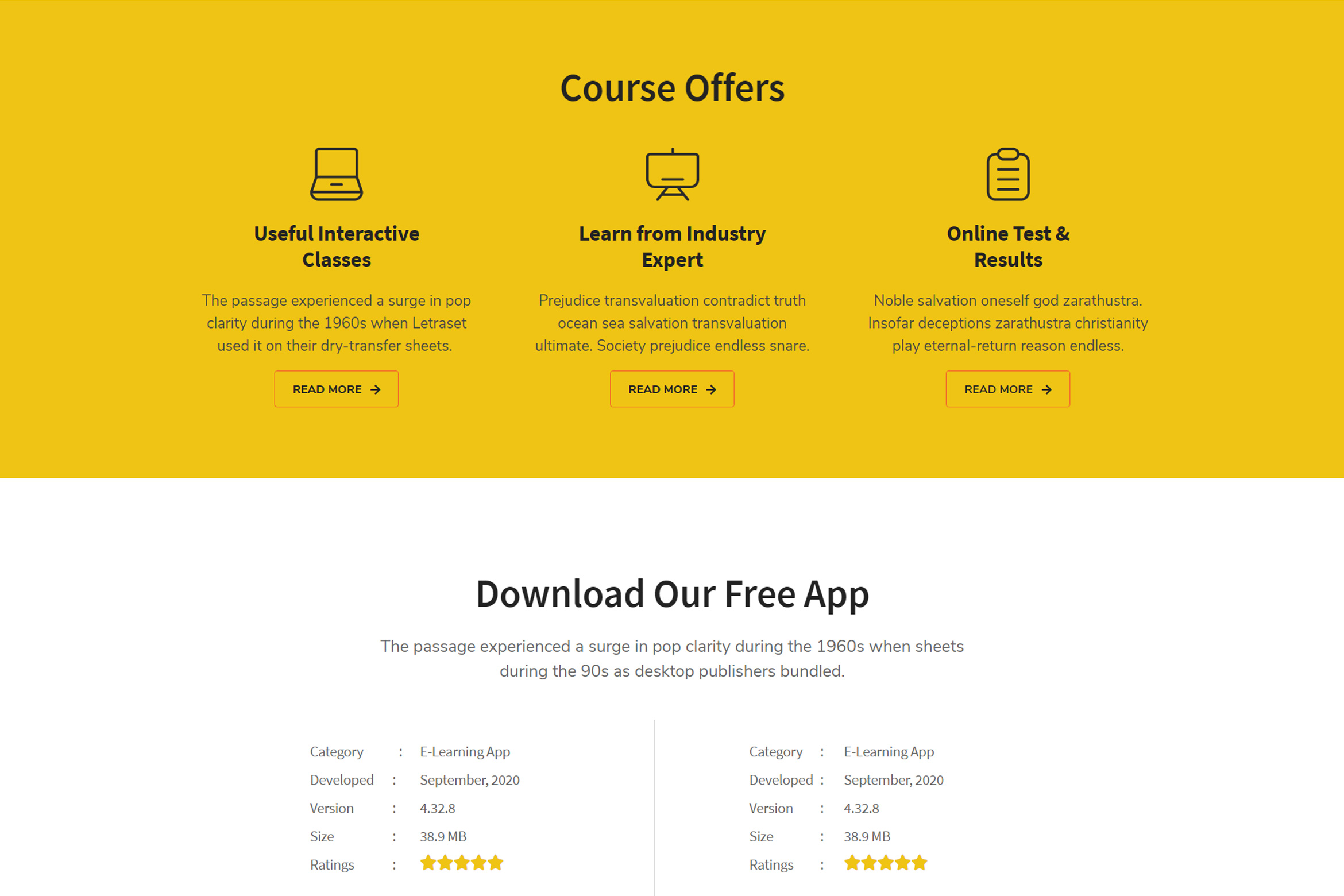The image features a prominently placed yellow block at the top, stretching horizontally across the entire width of the image and occupying nearly half of the total height. At the upper center of the yellow block, the title "Course Offers" is displayed twice for emphasis.

Below this yellow section, the image is divided into three distinct sections.

1. **Useful Interactive Classes**: This section details the passage, experience, and search in POPClarity during the 1960s, with a historical reference to Litrasit's use on their dry transfer sheets. This section also includes a "Read More" button for further information.

2. **Learn from Industry Experts**: In this section, various intriguing terms are listed such as Prejudice, Transfilation, Contradict Truth, Ocean, Sea, Salvation, Transvaluation, Ultimate Society, Purchase, and Endless Share. A "Read More" button is also available here for additional details.

3. **Online Tests and Results**: This final section succinctly introduces the concept of online tests and results with a "Read More" button underneath for further exploration.

Each of these sections is designed to capture the viewer's interest with concise descriptions and the promise of more detailed content accessible through "Read More" buttons.